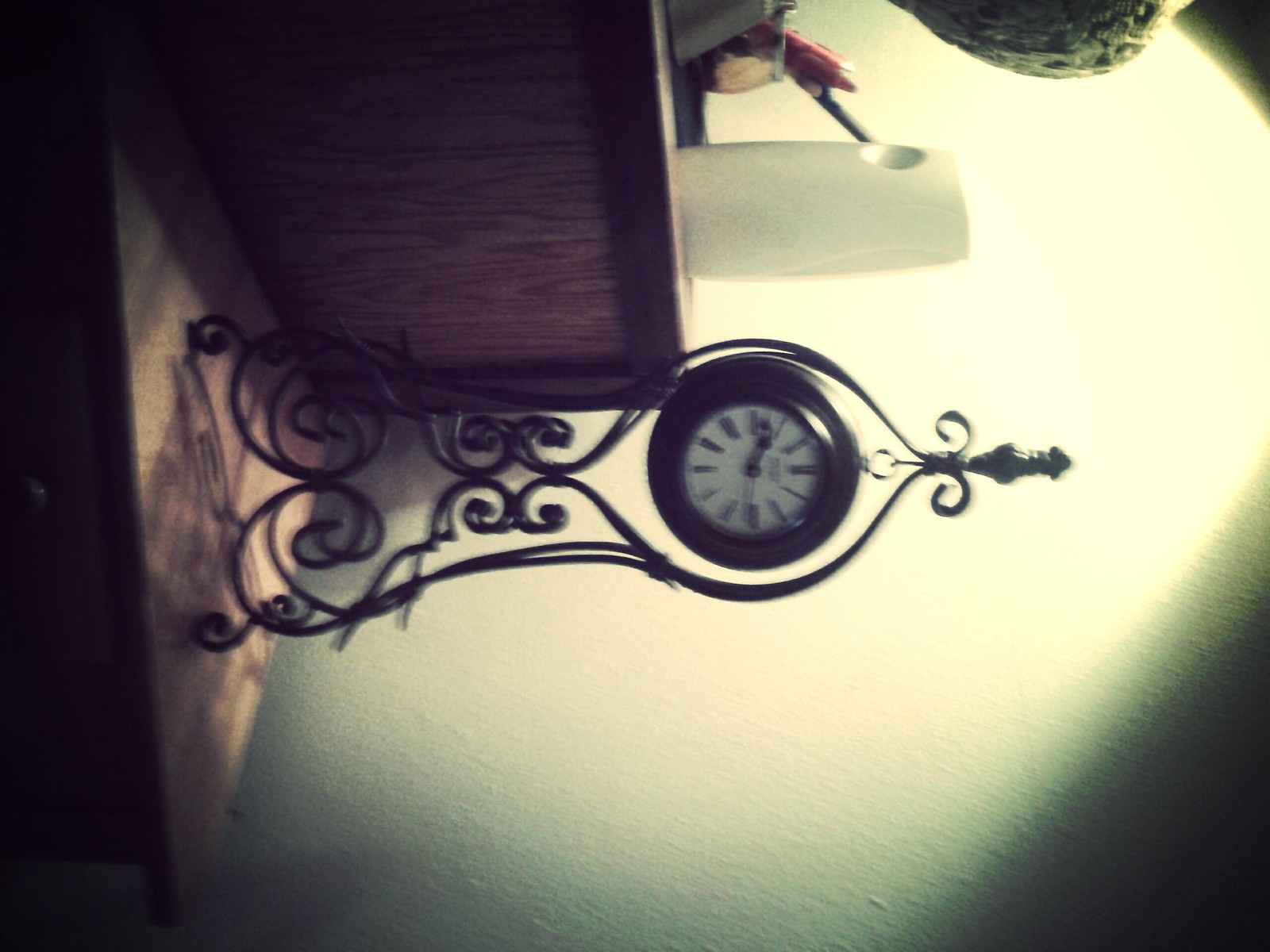In the image, there is a rustic wood grain table top, slightly tilted sideways, creating an intriguing angle. On the table rests an elegant black wrought iron stand, showcasing an intricate design. Suspended from the top of the stand is a classic clock, featuring a white background with bold black Roman numerals and matching black clock hands. Adding to the composition, another smaller, box-like wood grain table sits atop the main table. This secondary table supports a sleek white air purifier or sanitizer. The setting appears to be in a dimly lit room with white walls, illuminated by a single light source casting a gentle glow over the scene.